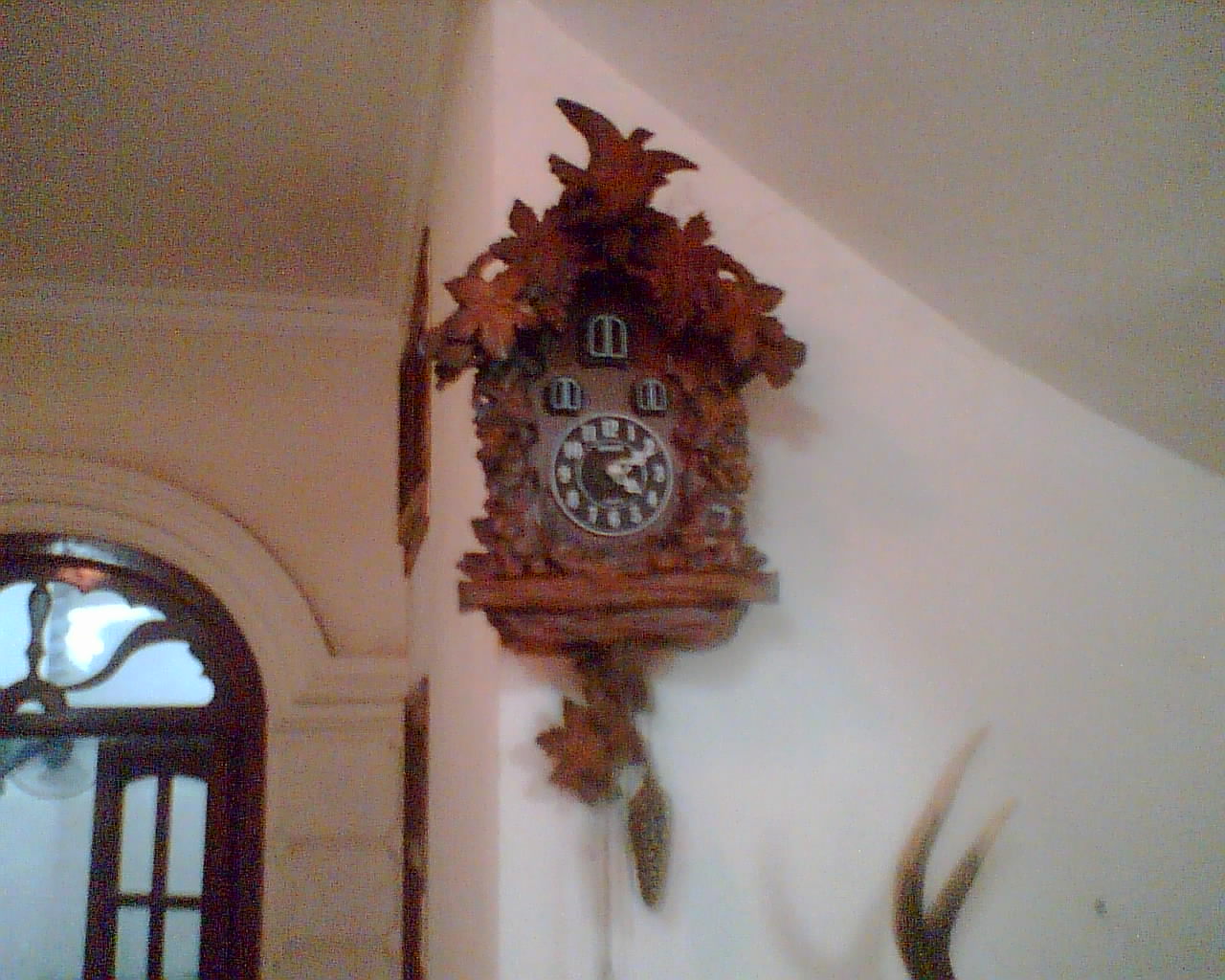A beautifully crafted, vintage cuckoo clock adorns the corner of a white wall. The clock is intricately decorated with elaborate wood carvings, featuring a charming bird, delicate flowers, and lush plant motifs. The clock face, finished in a striking silver color, displays both minute and hour hands, currently indicating the time to be approximately 4:10. Above the clock face, three ornately carved wooden windows are poised to open, ready to release the little cuckoo bird to chime. The clock is anchored by a decorative wooden weight, reminiscent of a grandfather clock's pendulum. In the background, the soft arch of a door or window adds a subtle architectural interest, enhancing the clock’s antique allure.